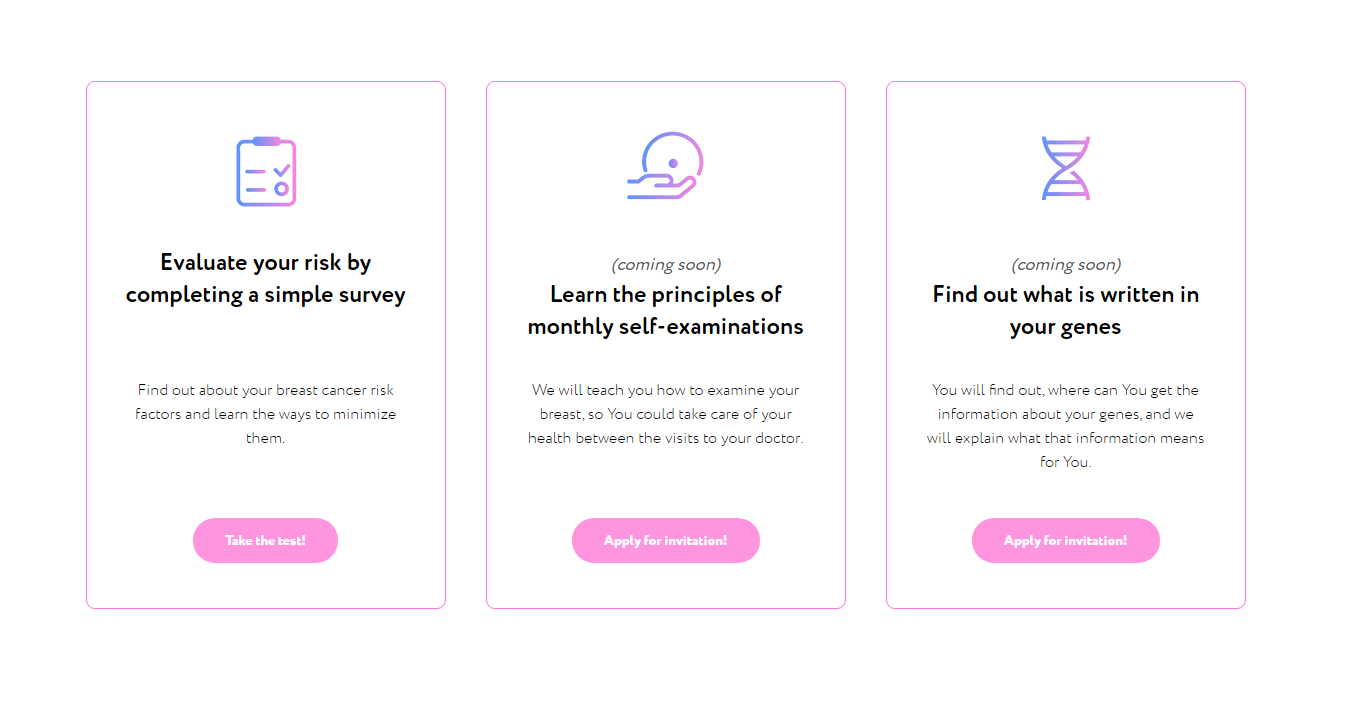The screenshot showcases a medical information website with three distinct panels, each designed to guide users through different health-related resources. 

- **Panel 1:**
  - **Icon:** A clipboard with a medical check symbol.
  - **Description:** "Evaluate your risk by completing a simple survey. Discover your breast cancer risk factors and learn ways to minimize them."
  - **Call to Action Button:** Light pink capsule with white text labeled "Start Survey."

- **Panel 2:**
  - **Icon:** A hand palpating a breast, symbolizing self-examination.
  - **Description:** "Coming Soon: Learn the principles of monthly self-examinations. We'll teach you how to examine your breasts effectively so you can maintain your health between doctor visits. Apply for an invitation."
  - **Call to Action Button:** Light pink capsule with white text labeled "Apply for Invitation."

- **Panel 3:**
  - **Icon:** A double helix representing genetic information.
  - **Description:** "Coming Soon: Discover what's written in your genes. Learn where to obtain genetic information and understand its implications for your health. Apply for an invitation."
  - **Call to Action Button:** Light pink capsule with white text labeled "Apply for Invitation."

Each icon features a gradient color scheme transitioning from a bluish-purple on the left to a pink on the right, while the overall design maintains a cohesive theme through the use of flat pink accents and white backgrounds.